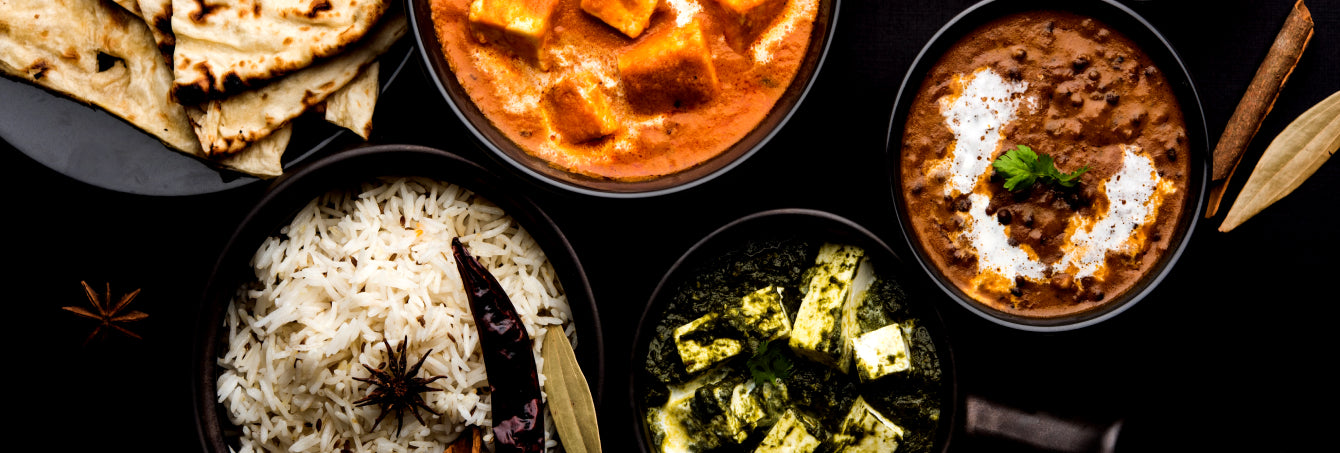The image depicts a tantalizing spread of what appears to be Indian cuisine, arranged on a dark table. The meal features several dishes served in black metal pots, viewed from a top-down perspective. The centerpiece is a pot of jasmine white rice, adorned with what looks like a long bay leaf and possibly a chili pepper. Adjacent to it, another pot contains creamy refried beans, garnished with a dried leaf that resembles oregano. A rich meat dish, likely butter chicken, is bathed in a light brown or orange sauce, occupying another pot. Complementing these are pieces of naan or pita bread, neatly stacked on a plate. One dish features what could be tofu, combined with green leafy vegetables, possibly spinach. Adding to the visual interest, the composition includes a cinnamon stick, a dried leaf, and a star-shaped wooden ornament in the upper left-hand corner, emphasizing the authentic and exotic presentation of the meal.